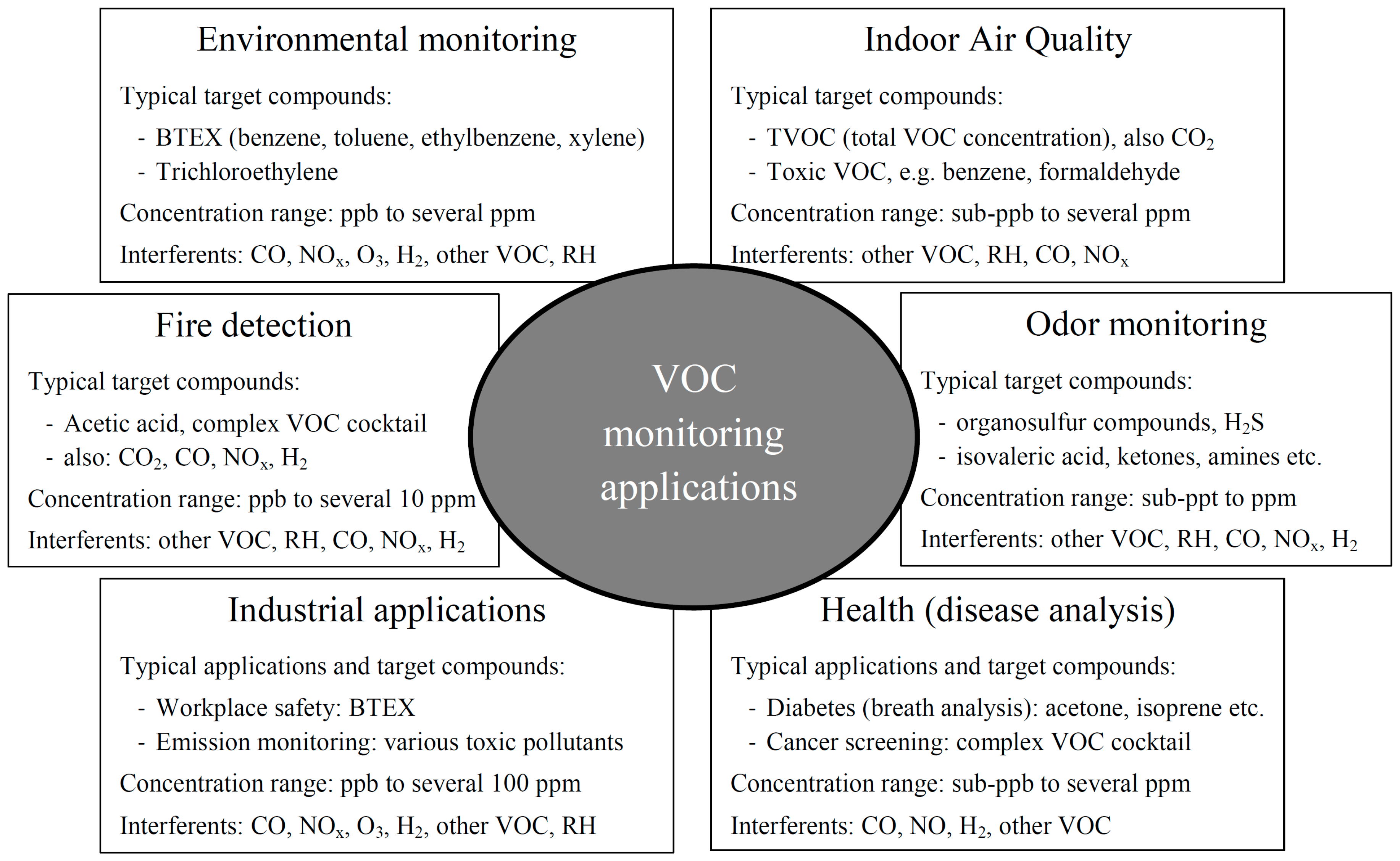This black-and-white infographic illustrates VOC Monitoring Applications at its core, emphasized by a central gray circle with white text. Encircling this central element are six detailed boxes that further elaborate on specific applications. At the 1 o'clock position is "Indoor Air Quality," which lists target compounds such as TVOC (Total VOC Concentration), CO2, and toxic VOCs like benzene and formaldehyde, with concentration ranges from sub-PPB to several PPM and potential interferences including other VOCs, RH, CO, and NOx. Continuing clockwise, the next box is "Odor Monitoring," followed by "Health Disease Analysis." Further on, "Industrial Applications" are specified, then "Fire Detection," and finally "Environmental Monitoring," which details target compounds like BTX (benzene, toluene, ethylbenzene, hexylene, trichloroethylene) with similar concentration ranges and interferences such as carbon dioxide, nitrogen, oxygen, helium, other VOCs, and NRH. Each box is framed with thin black lines, aligning and partially obscuring corners to fit the layout, giving it a textbook or guide-like appearance.